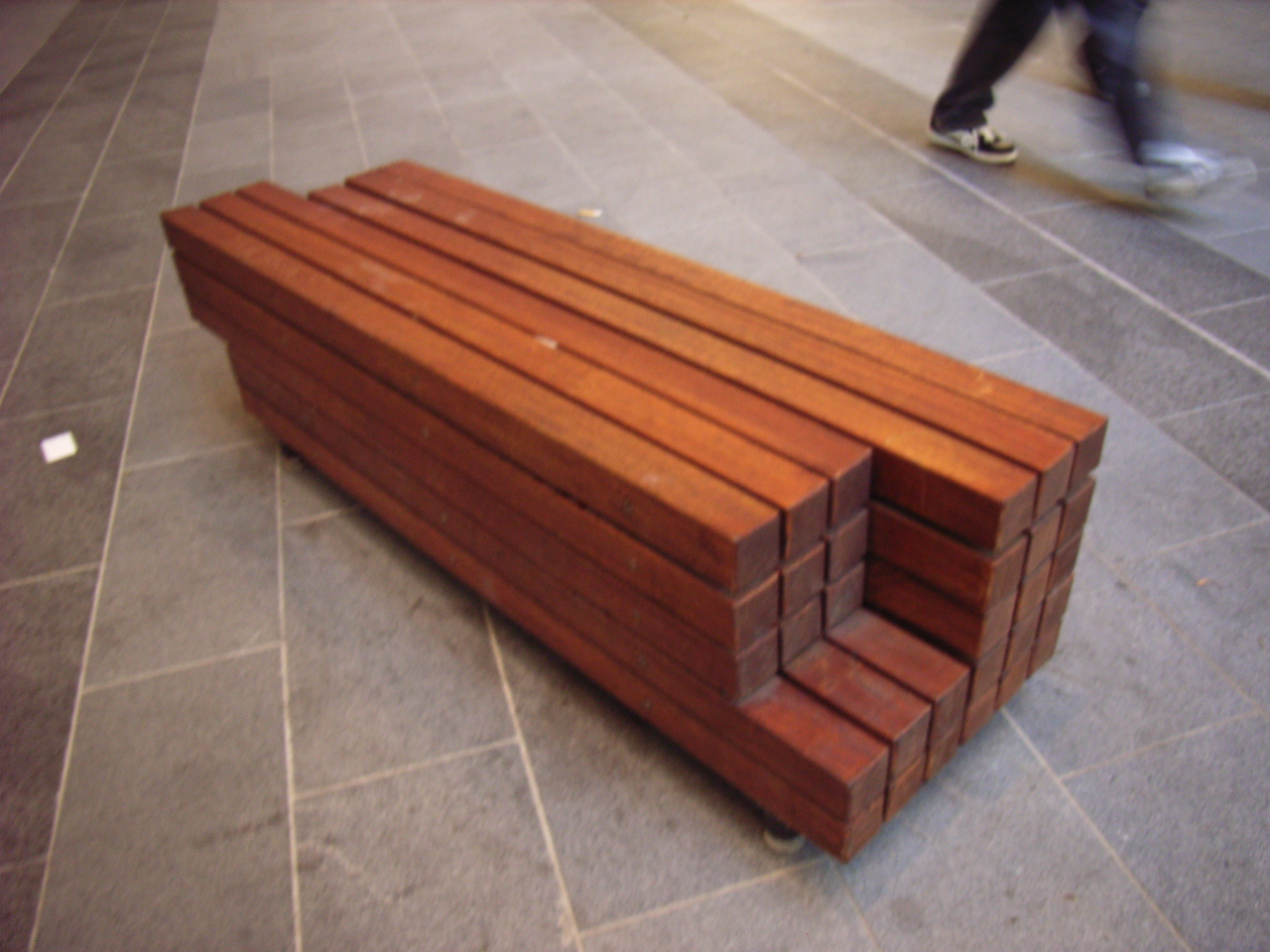A detailed photo reveals a meticulously arranged stack of rectangular cubic wood beams, resembling a deep red or dark cherry wood, evenly stained. The beams are stacked in a six-by-six formation, creating a cubic structure totaling thirty-six pieces. The top-left section of nine beams is slightly offset by about a foot. The entire setup rests on a light gray stone tile floor with darker gray tiles forming a border. The background shows the blurred legs of a man in motion, dressed in blue jeans and black-and-white sneakers, adding a dynamic element to the otherwise static composition.